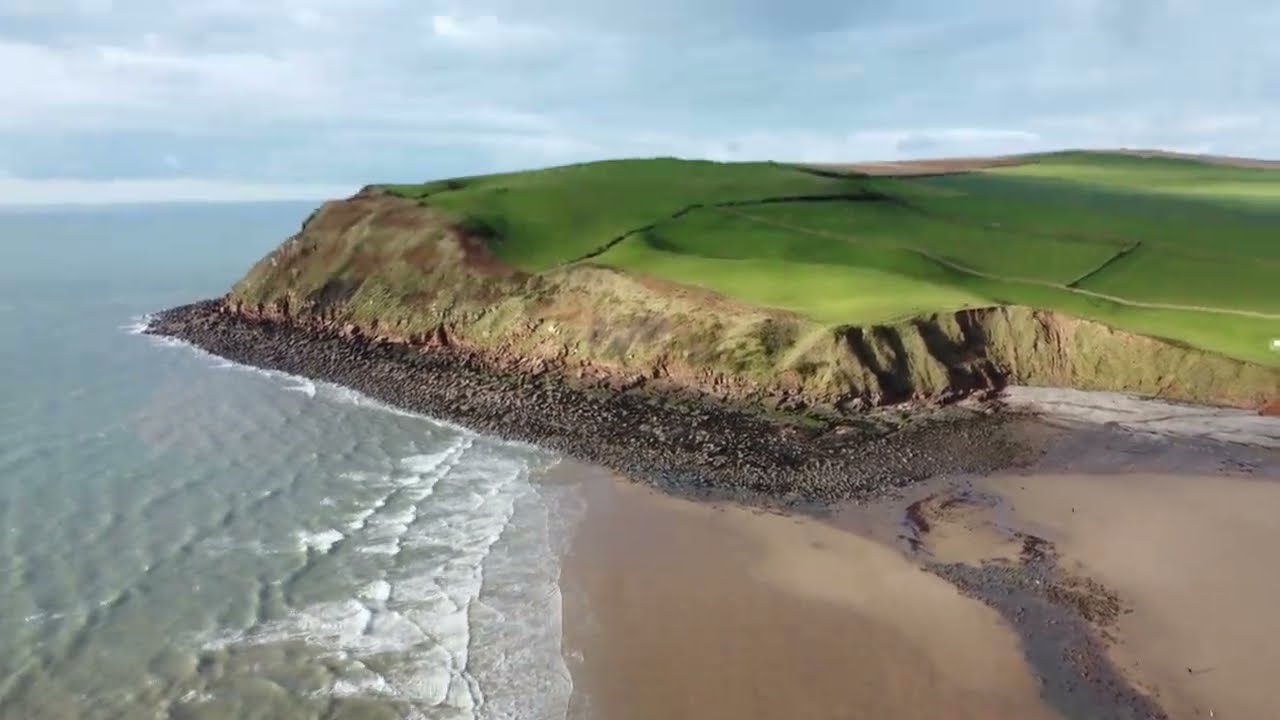The image is an aerial, computer-generated view of a coastal scene, showcasing a realistic yet digital aesthetic. At the top right of the image, there is a lush, green seaside plateau with subtle undulations on its flat top, blanketed with a smooth, almost painted-on layer of grass. This plateau has rocky sides, with sparse vegetation like moss adorning its steep, rugged slopes. The top of the image is dominated by a blue sky speckled with clouds, casting shadows on the landscape below. At the lower left corner, the terrain transitions into a turquoise ocean inlet, curving around the cliff. The foreground of the image features a beach with a mix of flat sandy areas toward the center and right, interspersed with rocky patches. The beach's left side merges into the clear blue water. The realism is diluted by a lack of fine details, making parts of the scene, such as the grass on the plateau, appear blurred and painting-like.